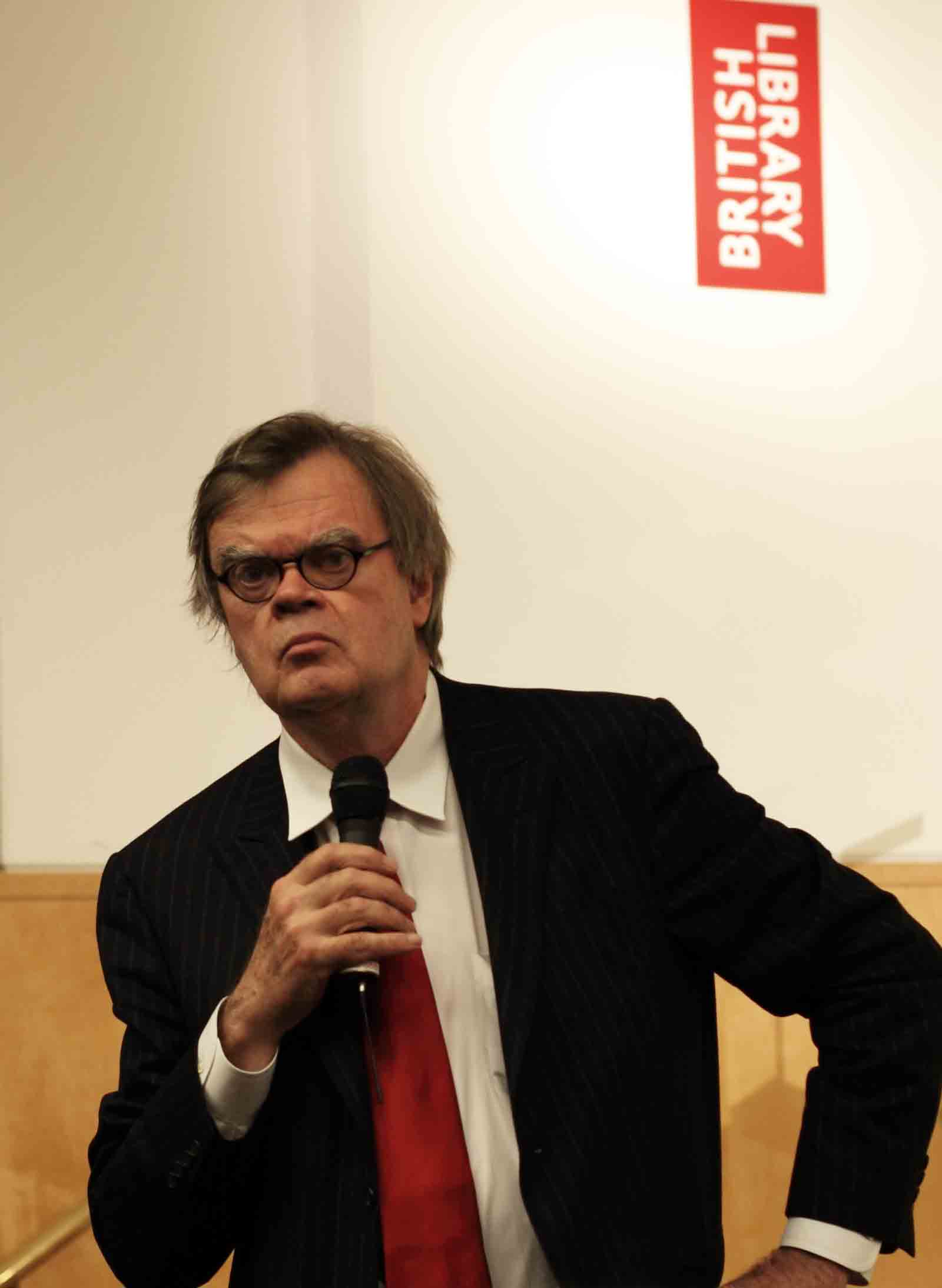A vertically oriented photograph captures a serious-looking Caucasian man in his fifties, standing from the torso up. He is dressed in a black pinstriped suit jacket, which is open to reveal a white collared shirt and a shiny red tie. His right hand, bent at the elbow, rests on his hip while his left hand holds a black microphone close to his chest. His grayish-brown hair is somewhat long and slightly bushy, and he sports small black-rimmed glasses. The man has a frown on his face and appears to be looking straight ahead, though slightly to the left.

In the background, the upper two-thirds of a white wall displays a red vertical rectangle with the words "British Library" in white capital letters, placed in an overlapping manner so that the words face each other. The lower part of the wall transitions into a mustard yellow wooden border. To the right, the wall has a lighter butterfly or double-triangle shape where light seems to be shining on it. The photograph captures a sense of formality and seriousness, possibly in a library or formal event setting.